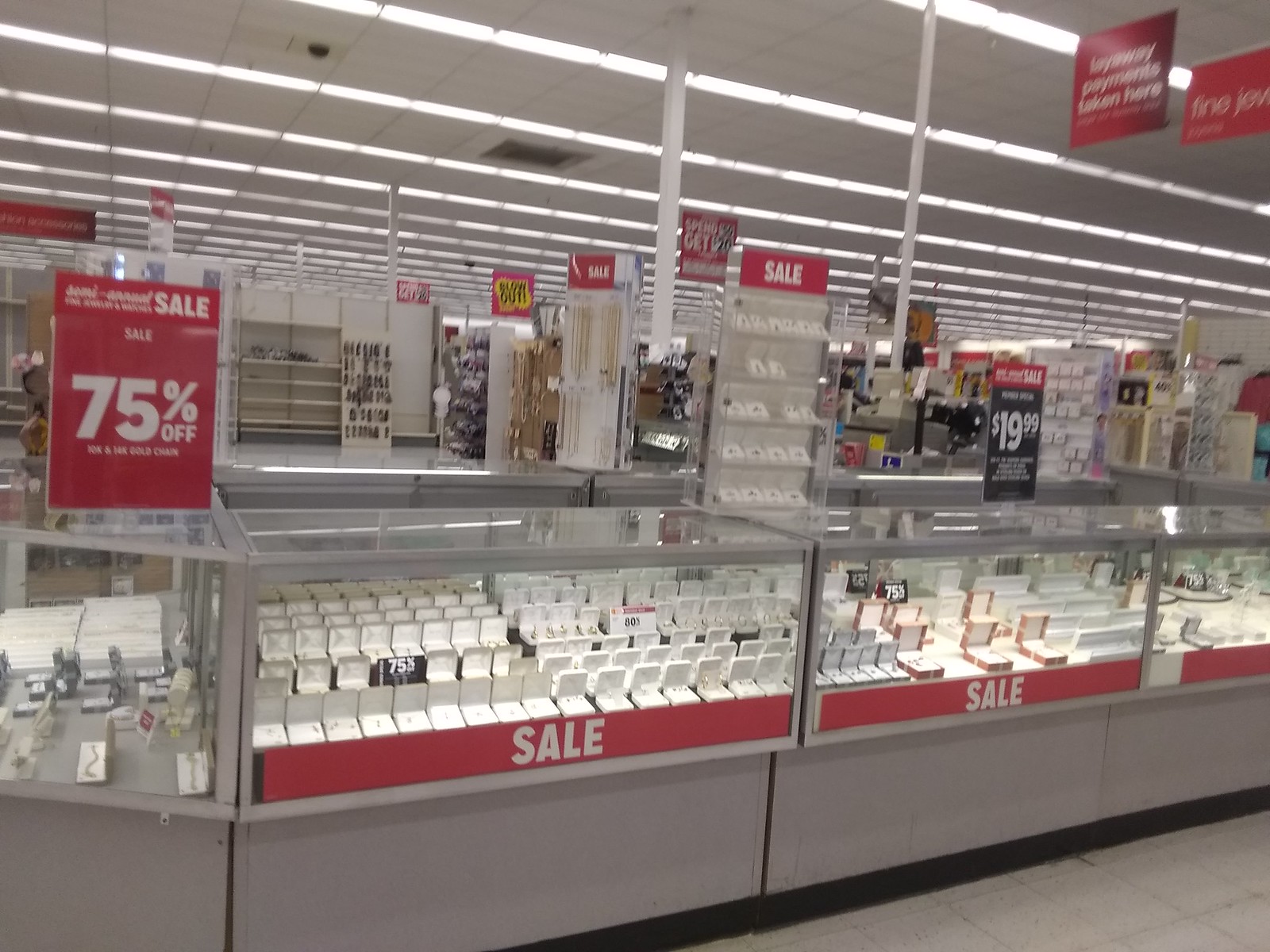The image depicts an inside view of a store featuring a jewelry sale. Dominating the scene are glass display cases filled with an assortment of fine jewelry, including rings, necklaces, earrings, and gold chains. Each case prominently features a red banner with "Sale" in white lettering at the bottom. Several black signs in the display announce a 75% off discount on 10 and 14 karat gold items, while a white sign advertises an 80% off deal. To the left, a large red sign further emphasizes the 75% off sale. In addition to the jewelry, a closer look reveals a variety of gold bracelets in the front left, and more gold chains in a rotating stand behind the counter. In the background, other sale items are visible, including various colored shirts in white, pink, and teal. Additional details include a price sign showing $19.99 and a note in the upper right corner indicating that layaway payments are accepted. The prevalent sale signage and abundance of jewelry highlight the store's promotional event.